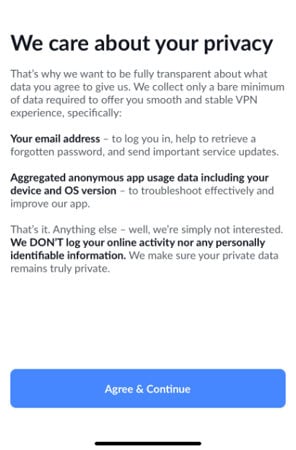Here is a detailed and cleaned-up caption for the image:

---

This section of a website addresses user privacy principles, prominently displaying the message "We care about your privacy" in the largest, boldest font. Below, the website communicates their commitment to transparency regarding data collection practices.

- **We collect only the bare minimum of data required to offer you a smooth and stable VPN experience.**
  - **Email address:** Used to log you in, assist with password retrieval, and send essential service updates.
  - **Aggregated anonymous app usage data**, including your device and OS version: This is collected to troubleshoot effectively and improve the app.

The message continues with an assurance:
- **That's it. Anything else, well, we're simply not interested.**
- **We don't log your online activity, nor any personal identifiable information.** 
- They emphasize their dedication to ensuring that your private data remains truly private.

At the bottom of the text, there's a blue, long rectangular button labeled "Agree and Continue" in white. The section concludes with a black bar running across the bottom of the page.

---

This caption summarizes the key points while providing a clear and detailed description of the privacy statement and call-to-action button.